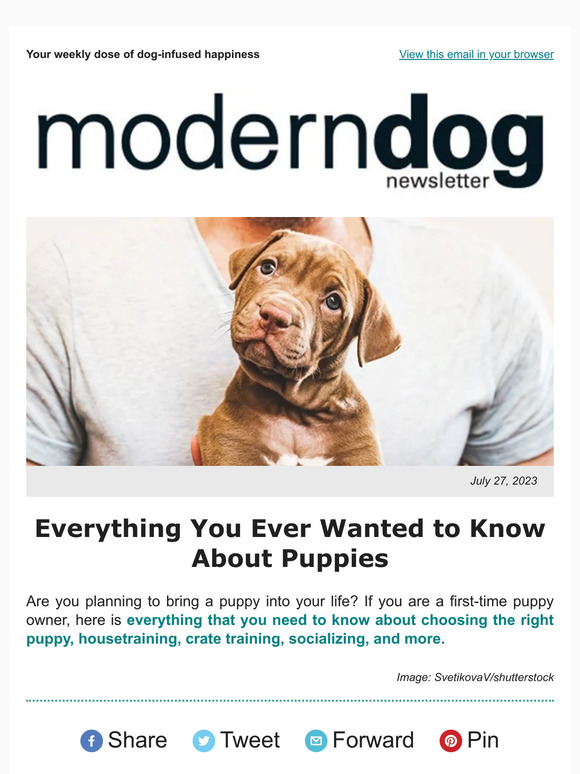The image features a minimalist design with a grey background and a prominent white block at the center, where all the details are contained. 

In the upper left corner of the white block, the text reads, "Your weekly dose of dog-infused happiness." To the right of this, there's a link labeled "View this email in your browser." The title "Modern Dog Newsletter" is prominently displayed, with the word "Dog" in bold.

Below this heading is a cropped image showing just the chest and shoulders of a person wearing a grey t-shirt, suggesting a male due to the visible neck. Dominating the foreground is an adorable brown puppy with its head endearingly cocked to one side. The puppy has hazel-colored eyes, floppy ears, and a cute little pink nose, resembling a hound dog breed.

Accompanying the image is a text that reads, "Everything you ever wanted to know about puppies. Are you planning to bring a puppy into your life? If you're a first-time puppy owner, here's everything you need to know about choosing the right puppy, house training, crate training, socializing, and more."

At the bottom of the white block are icons prompting social media interactions: "Share," "Tweet," "Forward," and "Pin."